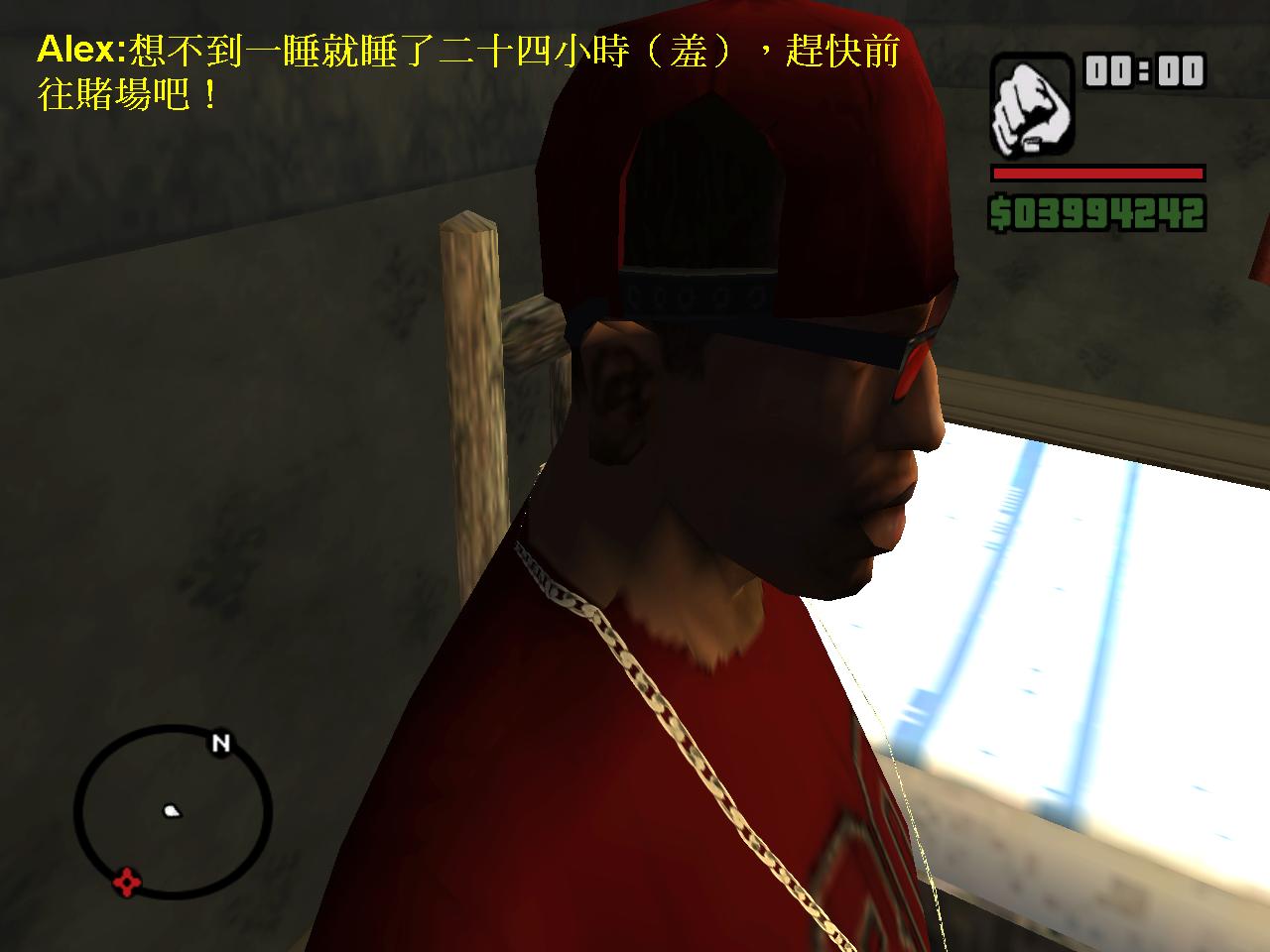The image is a screenshot from a video game, possibly from an older Grand Theft Auto series such as Vice City. The scene features a computer-generated African American man wearing a red baseball cap backward, black sunglasses with red lenses, a red t-shirt with the number 30 on it, and a long gold chain around his neck. The background shows him standing in a dimly lit room with dark gray walls and a window.

In the top left corner of the screen is the name "Alex" followed by Chinese text in yellow. The upper right corner displays a timer set to "00:00" next to an icon of a fist, indicating the current item being held in the inventory. Below this, there is a slim, rectangular red health bar. Further down is a dollar symbol followed by the amount of in-game currency, "03994242," in green with a black outline. The bottom left corner contains a mini-map showing the player's direction and quest objective.